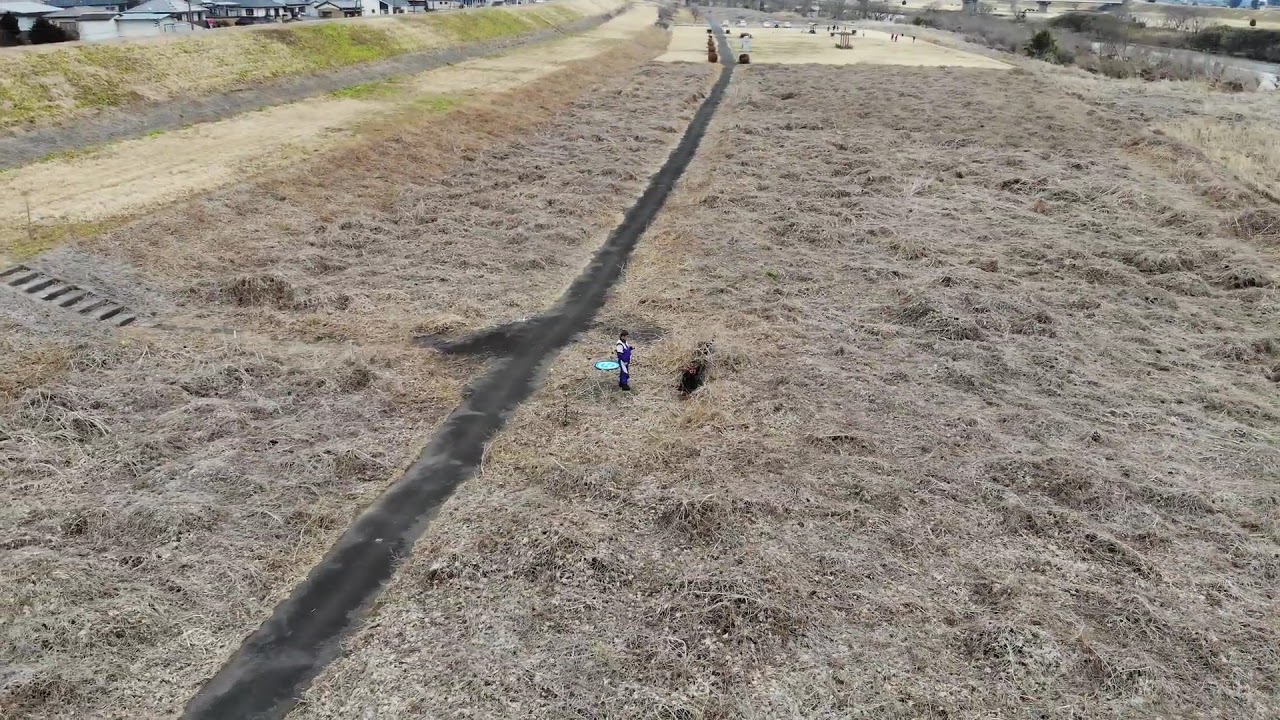The aerial photograph, likely taken by a drone, captures a desolate landscape dominated by a vast, overgrown field of dying, brown grass, suggesting a drought-stricken area. At the heart of the image stands a man dressed in a purple tracksuit, positioned near an old sewer lid in the otherwise barren field. Stretching across the field is a barely discernible dirt path, possibly created by a tractor. To the left of the man, there's an asphalt pathway for walking or cycling, which leads to a set of stone steps going up to a dirt or gravel walkway on an elevated level. A thin stream of water winds through the field, adding to the sense of dryness and neglect, potentially hinting at a dried marsh. Adjacent to the field, on the right side, runs a road, and further up the picture, a park can be seen where people are playing despite the parched surroundings. To the left, the scene includes a suburban neighborhood with a cluster of houses on the outskirts, under an overcast sky that complements the overall bleak and dry atmosphere.